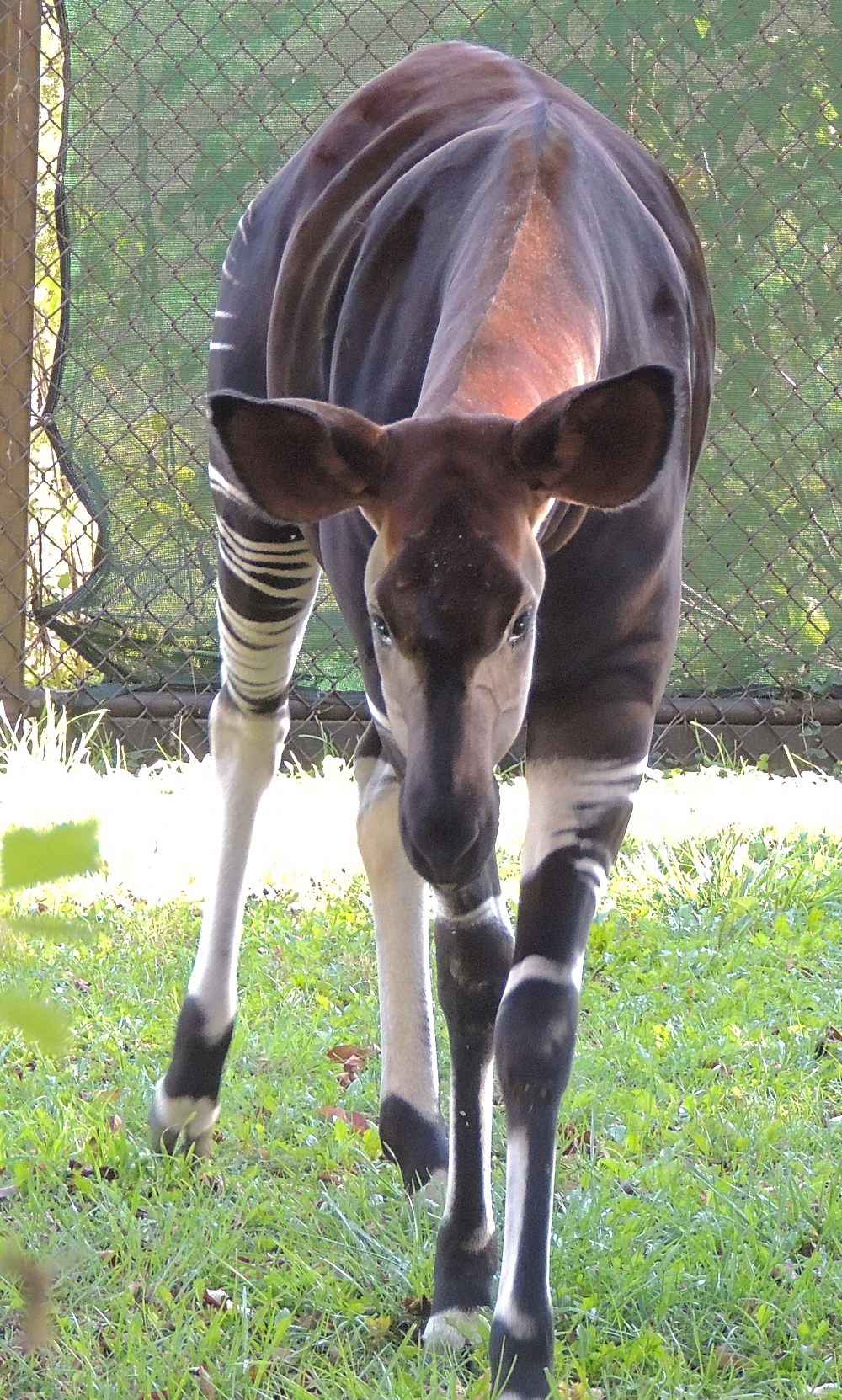This color photograph in portrait orientation captures a large, exotic mammal resembling a zebra with special photographic effects on its front half, transforming it to look like a dark-colored horse with a slightly pointed muzzle and large round ears. The animal is positioned centrally and appears to be walking towards the viewer in a grassy field interspersed with clover and dandelions. The image's background features a chain-link fence with a green shade fabric, and there are no people or additional objects present. The colors predominantly include brown, green, yellow, white, and black, highlighting the animal amidst the grass and the fenced backdrop, possibly suggesting a zoo setting or use in an online article about animals.